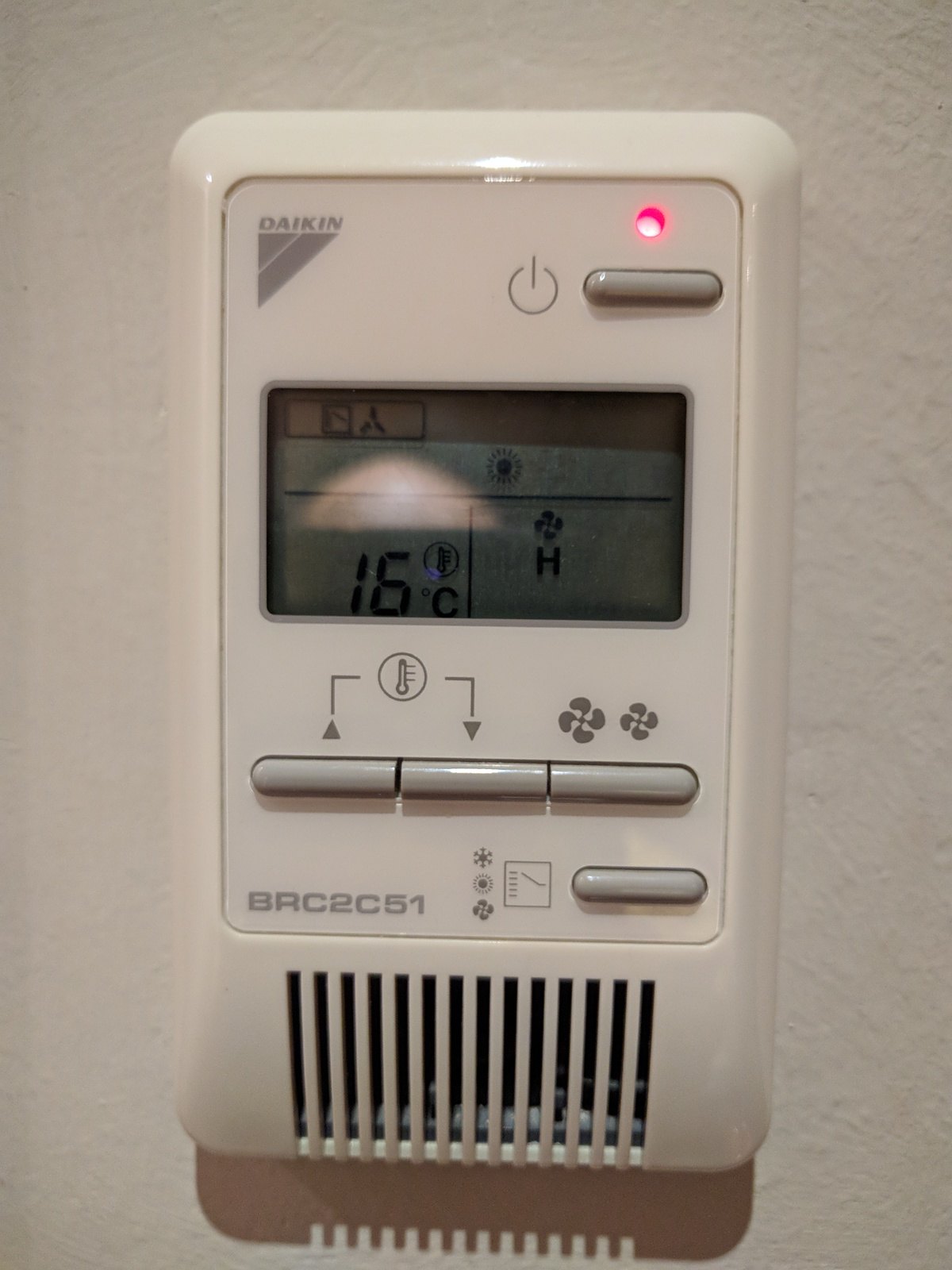This photograph captures a Daikin thermostat mounted on a pristine white wall. The thermostat, a sleek rectangular device, features a small, rounded rectangular power button at the top, illuminated by a red light indicating it is on. The display screen shows the current setting of 16 degrees Celsius, with the heat mode active, as depicted by a corresponding symbol. A reflection of a light behind the photographer is faintly visible on the screen.

Beneath the display are three buttons aligned horizontally: two marked with arrows for incrementing or decrementing the temperature, and a third button for adjusting the fan speed. At the bottom of the thermostat is a row of symbols—a snowflake, a fan, and a sun—likely representing modes for cooling, fan operation, and heating. Below these symbols is a vent, characterized by several vertical slits, which appears to facilitate airflow through the unit.